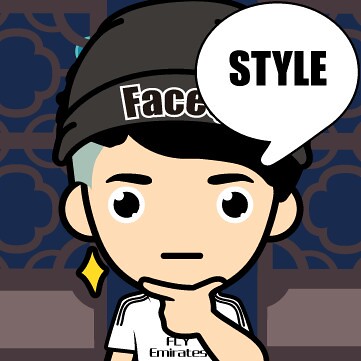This full-color cartoon illustration, drawn with bold computer graphics-style outlines, features a boy with light skin, standing in front of a wall adorned with blue and gray floral patterns. The boy has a neutral expression, with his mouth as a straight line, and large, expressive eyes consisting of white half-circles inside black pupils. He has black hair with a section shaved light blue. He's wearing a dark gray ski cap that says "face" on its rim, although part of it is obscured by a speech bubble. The speech bubble, positioned on the right side of the image, contains the word "style" in bold, black capital letters. The boy is dressed in a white t-shirt that says "Fly Emirates" with black stripes on the shoulders. He is depicted holding his hand up to his chin, with his thumb and index finger extended, as if in a thinking pose. Additionally, he wears a diamond-shaped yellow earring on his left ear, which adds a unique touch to his appearance. A yellow star is situated next to his face, completing this thoughtfully crafted avatar-like character.